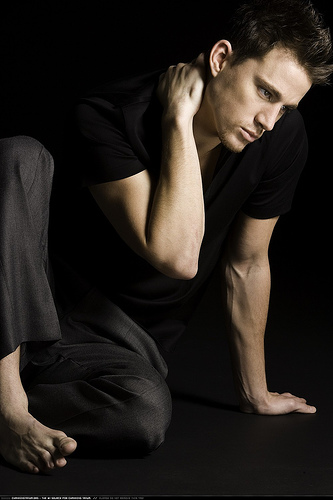In this detailed color photograph, a barefoot man is sitting on an indistinct black surface, seamlessly blending into a matching black background, creating the impression of a black void. The man is wearing dark gray dress pants and a slightly shiny black short-sleeve t-shirt. His left hand is extended to the ground for support, while his right hand is brought up to his neck, giving the impression of either wringing or scratching. He sits with his right knee bent up. The man has dark brown, short yet thick and spiky hair, and his face is clean-shaven. His serious expression is directed downward and to the lower right corner of the image, towards an off-screen point. The white text, blurred and nearly illegible, spans five to six words in the bottom left of the photograph.